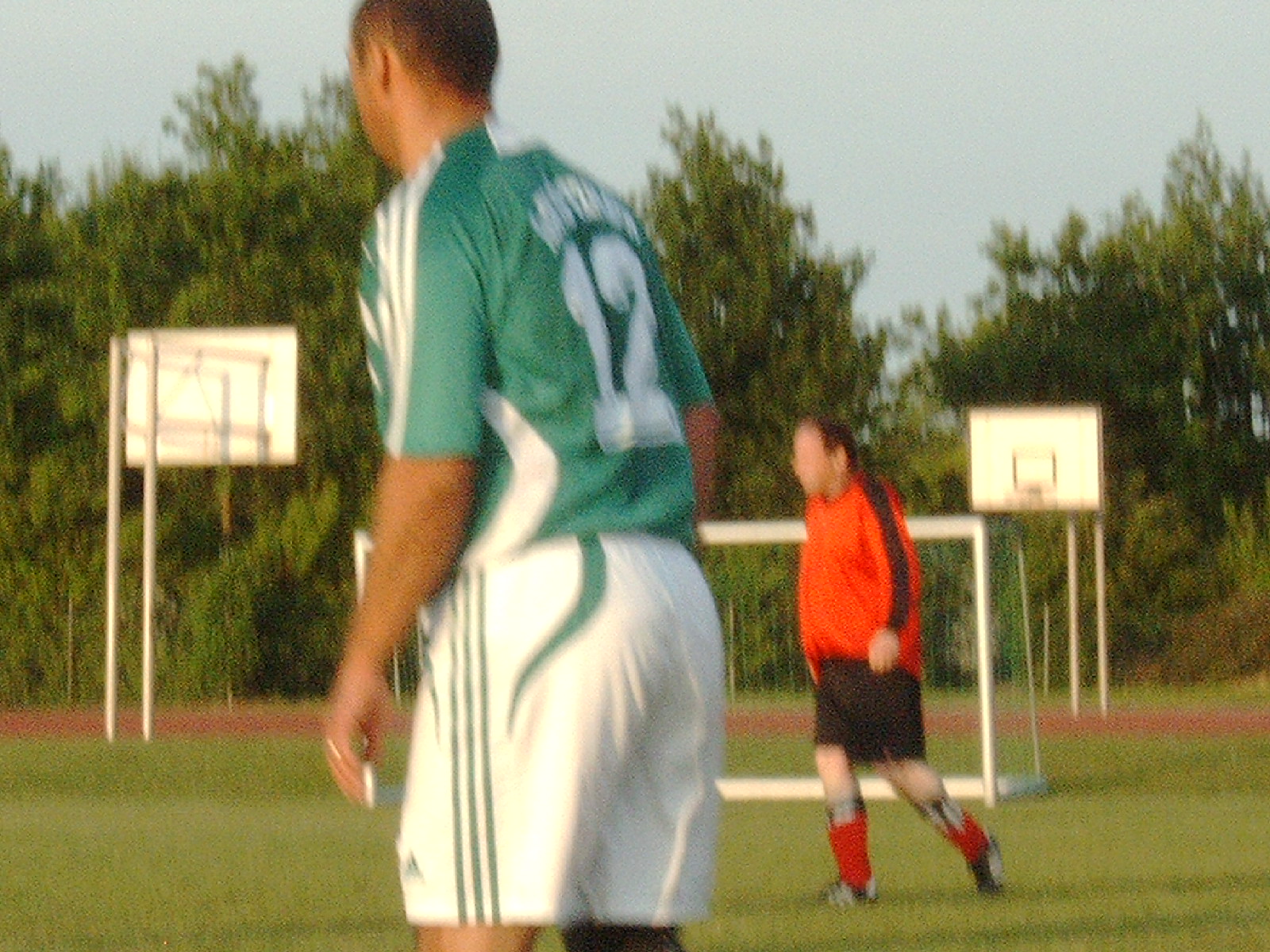In this outdoor scene likely set at a high school sports field, two soccer players are captured in action on a slightly blurry photograph. In the foreground stands an African American player wearing a green jersey with white stripes on the arms and the number 12 on his back, paired with white shorts featuring green stripes along the sides. Further back near the goal is another player in a red long-sleeve jersey with black pants and red socks. The scene is illuminated by a somewhat grayish sky, suggesting it might be late afternoon or early evening, potentially in the fall. In the background, there is a basketball court with hoops at each end and a line of trees framing the scene, completing this dynamic sports environment.